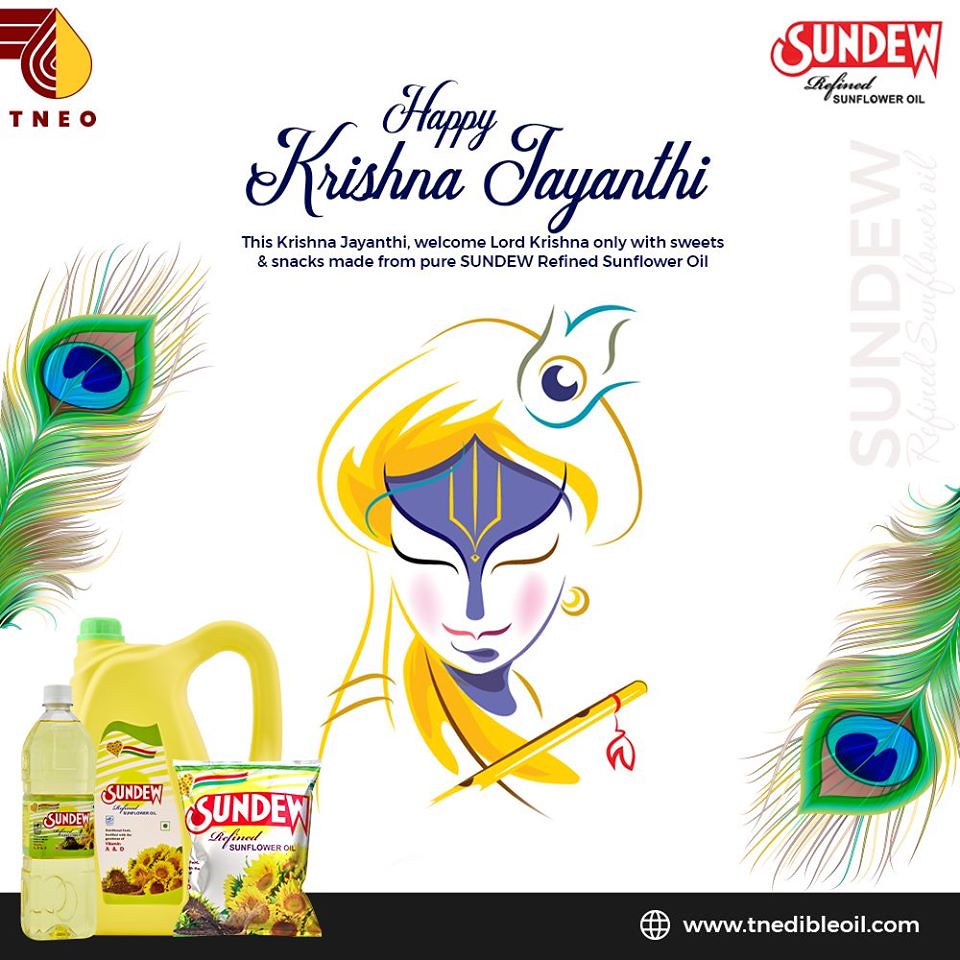This square digital advertisement features a pristine white background. Dominating the top left corner is a teardrop-shaped logo, half brown and half yellow, with the letters T-N-E-O in brown capital letters. In the top right corner, a red logo reads "Sundew" in white font, with "refined" in black cursive below and "Sunflower Oil" in capital letters.

Central to the image is a blue cursive inscription that reads "Happy Krishna Jayanthi," followed by the message in simple font: "This Krishna Jayanthi welcome Lord Krishna only with sweets and snacks made from pure Sundew refined Sunflower Oil." Beneath this text stands a vibrant, purple and gold illustration of a Hindu deity flanked by two adorned peacock feathers—one on the left and one on the right.

Adjacent to the deity is a detailed figure of a woman adorned in a yellow and purple headdress, gold earring, red lipstick, and a delicate peacock feather on the right side of her head. At the bottom left of the advertisement, various Sundew oil products are showcased: one clear bottle with a lid, another yellow pour bottle, and a package of sunflower seeds, representing the diverse offerings of the brand.